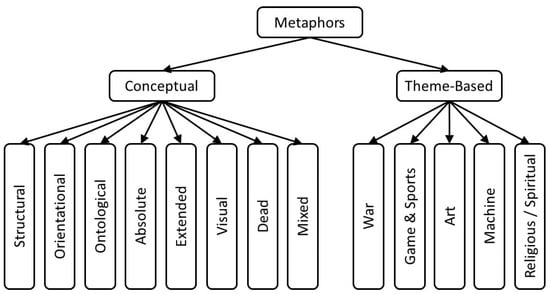The image is a minimalistic black-and-white flowchart on a white background, detailing the meaning and use of metaphors within a literary context. At the top, the word "Metaphors" is prominently displayed in a horizontal rectangle. Two arrows branch downward from this rectangle, pointing to the categories "Conceptual" and "Theme-based," which are also in horizontal rectangles. 

Under "Conceptual," there are eight subcategories arranged in vertically oriented rectangular boxes: "Structural," "Orientational," "Ontological," "Absolute," "Extended," "Visual," "Dead," and "Mixed." Similarly, from the "Theme-based" category, arrows point to vertically oriented rectangles titled: "War," "Game and Sports," "Art," "Machine," and "Religious/Spiritual." This clear and organized chart effectively summarizes different types of metaphors in literature, using a straightforward visual format with vertical text for subcategories and horizontal text for main categories, all depicted in black font.